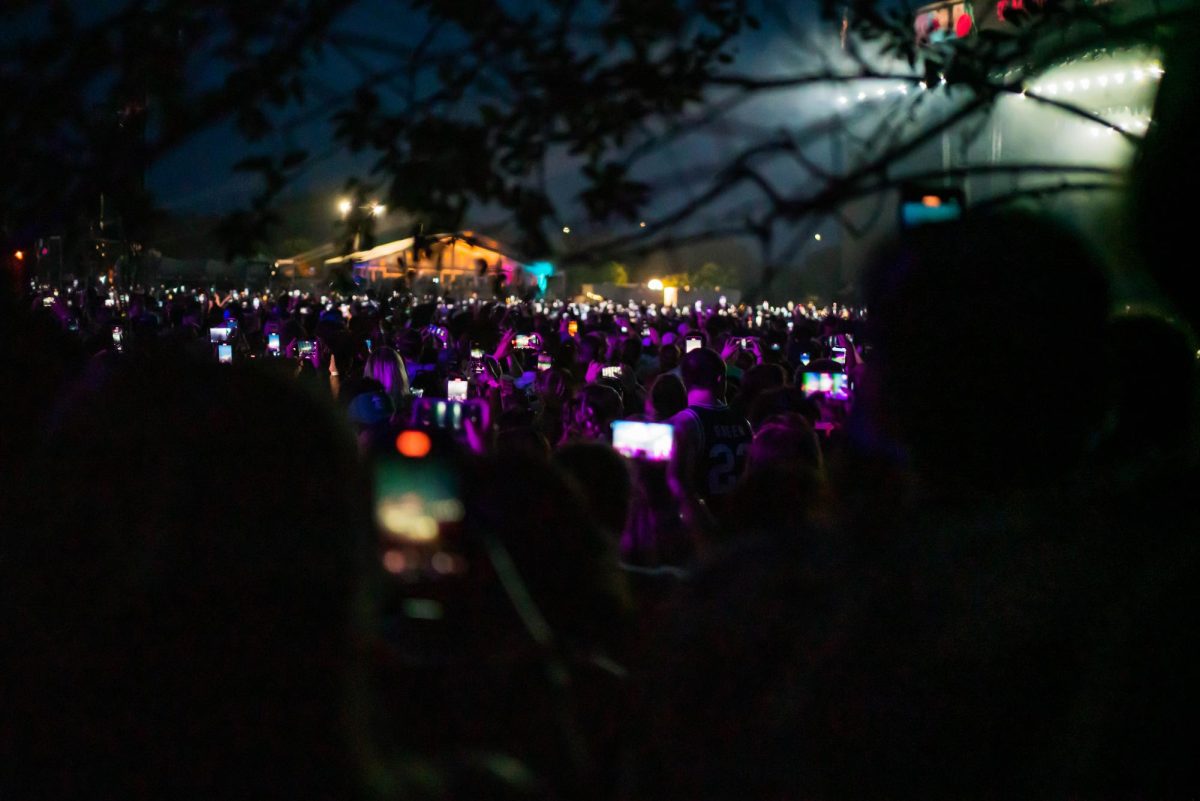This photograph captures the vibrant atmosphere of an outdoor concert at night. The scene is dominated by a large crowd of people, all facing a stage and holding up their cell phones to record the performance. The multitude of phone screens creates a kaleidoscope of light amidst the darkness. The audience is bathed in a purplish glow from the stage lights, which adds a surreal and almost ethereal quality to the image. To the right, the darkness is punctuated by the silhouette of tree branches, adding an element of natural framing to the scene. In the background, a peaked-roof house can be seen, illuminated by the pink and blue lights that pepper the event. Stadium lights on the right side provide additional illumination, casting a mixture of tan, red, and white tones across the night sky. The overall color palette of the photograph is a blend of black, purple, blue, and white, encapsulating the essence of a lively, nocturnal celebration.